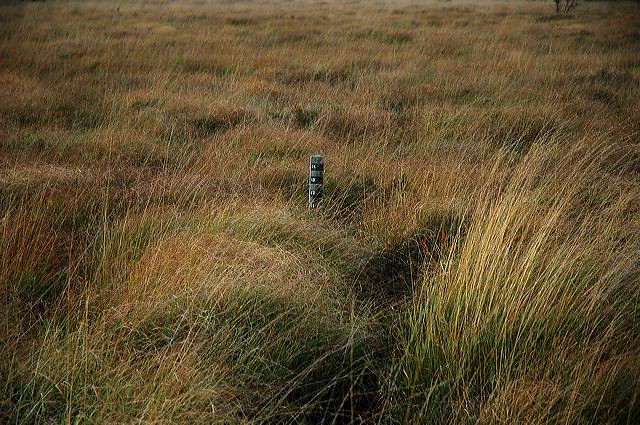The image captures a sprawling, overgrown grassy field under the bright daytime sun, with thick, tall shoots of grass dominating the landscape. The grass varies in color, predominantly exhibiting shades of green and yellow, with patches of brown and dried-up areas hinting at a possible fall setting. The dense grass, in some parts, creates shadowed areas that resemble frizzy hair. Amidst this wild field stands a solitary, gray post that resembles a vertical ruler or a meter, marked by black and white text. In the top right corner, a withering bush or tree adds to the scene's untamed and somewhat neglected appearance. The field stretches as far as the eye can see, emphasizing the overgrown and uninhabited nature of the location.